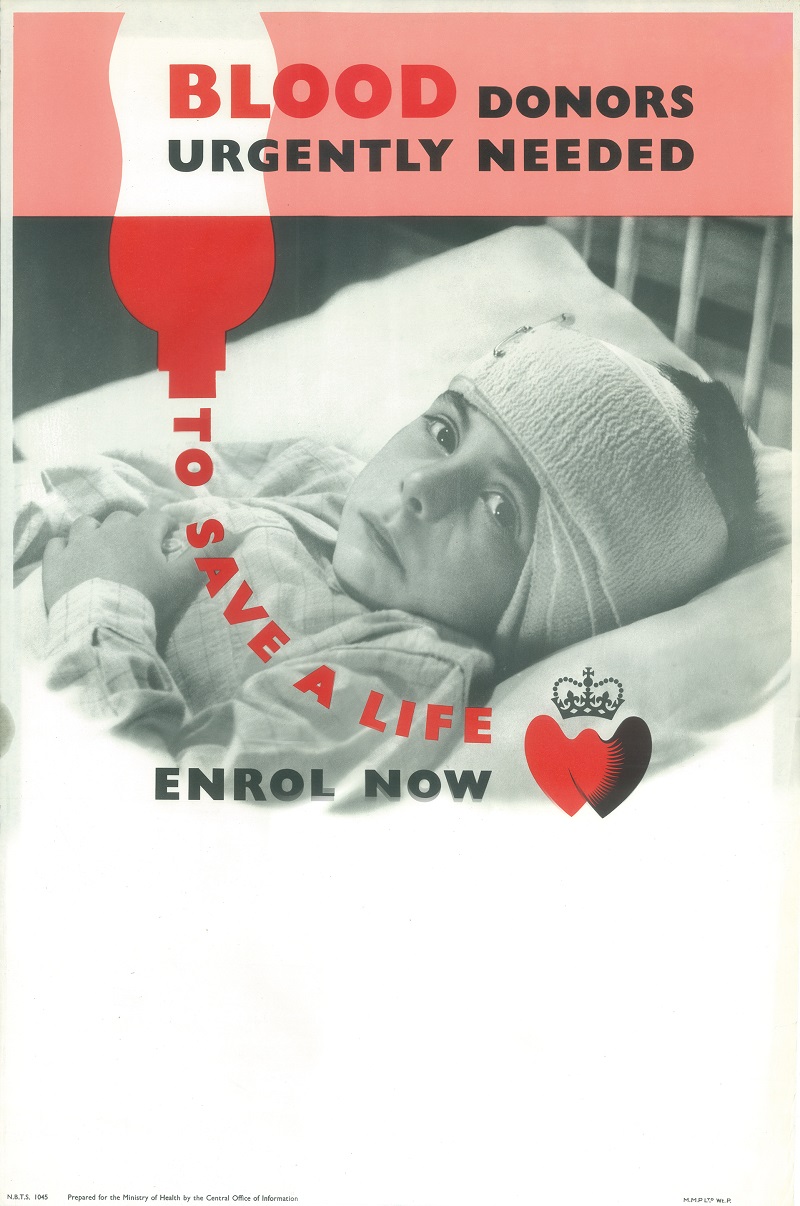This recruitment poster for blood donors depicts a compelling black and white photograph of a young boy, likely around 7 to 10 years old, lying in a hospital bed. The boy, dressed in a white hospital gown, has his head heavily bandaged with white gauze and safety pins securing the wrapping. He is gazing directly into the camera with a solemn expression, amplifying the urgency of the plea. The image is older, suggesting it might have been created decades ago.

Dominating the top portion of the poster is a pink rectangle with the word "Blood" in bold, large red letters, followed by "Donors" and "Urgently Needed" in black. A cartoon-like IV bag is illustrated behind the word "Blood," transitioning from white at the top to red at the bottom, symbolizing blood collection. Just below the IV bag, the red text states, "To Save a Life," followed by "Enroll Now" in black, though the word "Enroll" is spelled "E-N-R-O-L," indicating a potential non-U.S. origin. 

At the bottom right corner, a logo representing a red heart and a black heart, with a crown hovering above them, emphasizes the noble cause. Additionally, there is very fine print at the bottom, which reads, "Prepared for the Ministry of Health by the Central Office of Information," alongside possibly some letters and numbers, such as "NBT-1045," which are largely illegible due to their minuscule size.